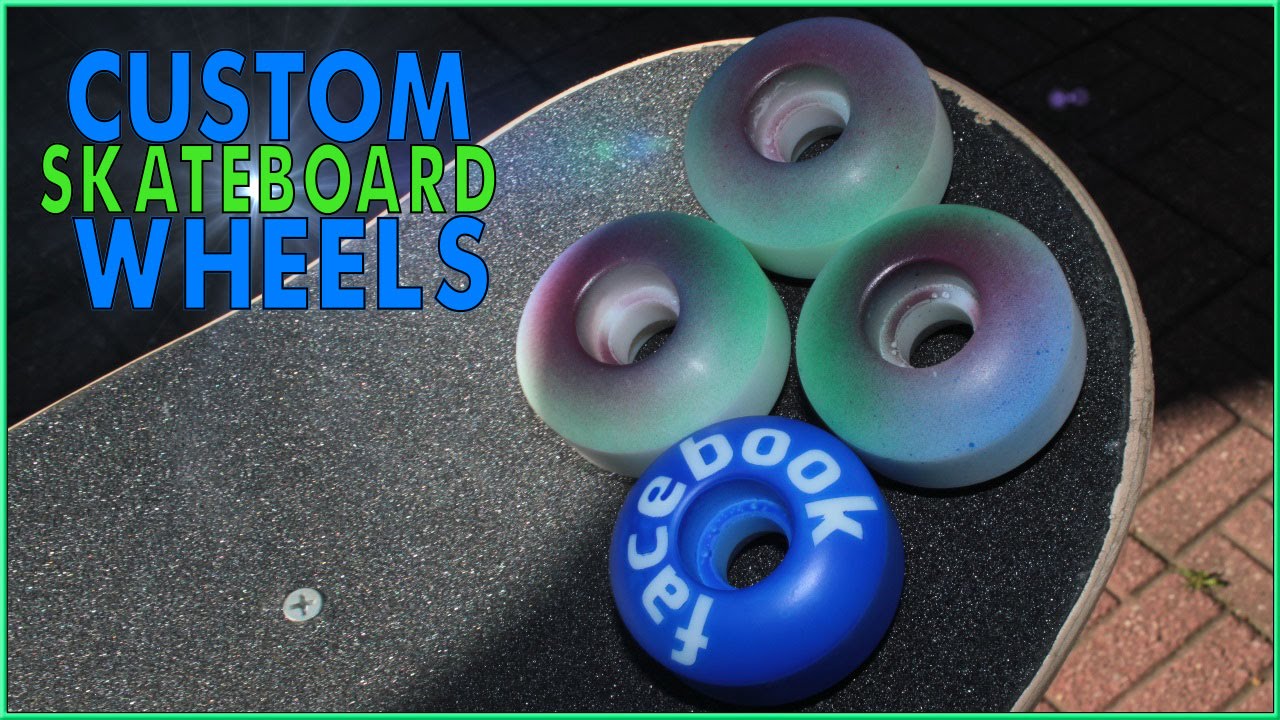The image showcases a worn, well-loved skateboard, featuring black grip tape on its deck. Positioned on the nose of the skateboard in a diamond shape are four custom skateboard wheels. Three of the wheels are white, while the fourth one stands out in blue, emblazoned with the text "Facebook" in white, echoing its hue. Overlaying the image is a vibrant advertisement message in all caps: "CUSTOM SKATEBOARD WHEELS," with the words "CUSTOM" and "WHEELS" in blue, and "SKATEBOARD" in green. The background reveals a brick floor, adding to the vintage and rugged aesthetic of the scene. Overall, this advertisement emphasizes the ability to personalize skateboard wheels, using the Facebook-branded wheel as an example.